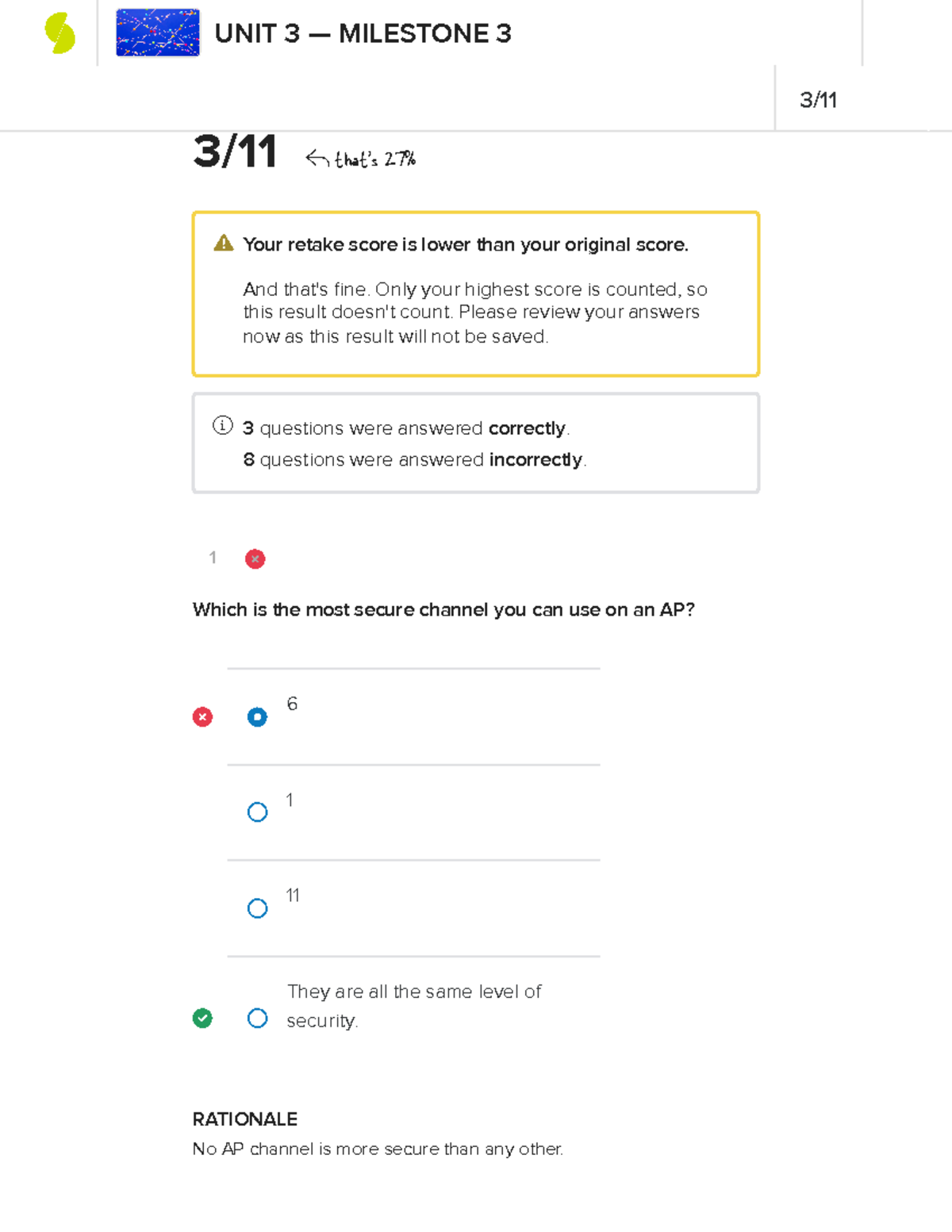**Screenshot of Web Page: Unit 3, Milestone 3 - Assessment Results**

At the top of the image, there is a white banner featuring two icons. The first icon consists of two offset halves of a light green circle, and the second icon is a blue rectangle with lines and dots in various colors. To the right of these icons, "Unit 3 / Milestone 3" is displayed in black text. Below this header, the text "3 / 11" is shown, indicating progress. A note beside this, written in small handwriting, states, "That's 27%".

Beneath this section, a yellow outlined box contains a warning message adjacent to a triangle icon with an exclamation point inside it. The warning reads: 

"Your retake score is lower than your original score and that's fine. Only your highest score is counted, so this result doesn't count. Please review your answers now as this result will not be saved."

Further down, a gray outlined box provides a summary of the test performance: 

"3 questions were answered correctly. 8 questions were answered incorrectly."

Below this summary, a specific question from the original test is shown. The question asks: 

"Which is the most secure channel you can use on an AP?"

Three answer choices are provided: 6, 1, and 11. The selected answer, "6", is highlighted with a white mark inside a blue circle. An incorrect icon (X within a circle) is displayed to the left of this answer, whereas a green checkmark is next to the correct answer, indicating "They are all the same level of security."

Underneath this question, the explanation ("Rationale") is provided:

"No AP channel is more secure than any other."